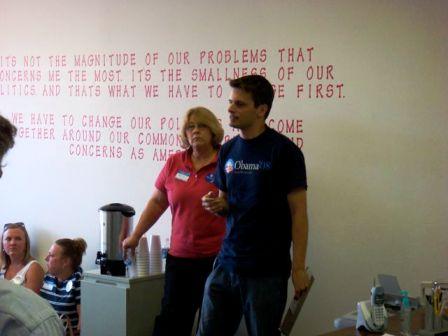In this color photograph, a man and a woman stand in the center of the image in front of a white wall with red writing. The woman, who has short blonde hair and glasses, is wearing a red button-down, short-sleeved polo shirt and black pants. She has a name tag on the left side of her chest. Next to her stands a taller man with dark brown hair, wearing a blue Obama t-shirt and blue jeans, suggesting his support or volunteer status for Obama's campaign. To the left of the woman, there is a small cabinet with a coffee pot and two stacks of disposable cups on top. The incomplete writing on the wall behind them reads, "It's not the magnitude of our problems that concerns me the most, it's the smallness of our politics, and that's what we have to... together around our common concerns as Americans." On the bottom left, you can see two females seated, possibly on the floor, and there is also an old landline phone and various other objects.